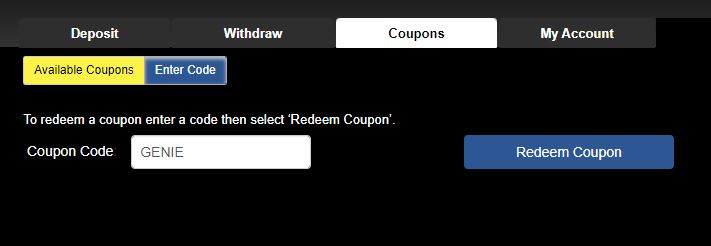The image appears to be a partial screenshot of a user interface on a black background. At the top of the screen, there is a horizontal gray stripe spanning almost the entire width, terminating about three-quarters of the way across. Towards the right end of the stripe, there is a smaller segment that runs to the edge of the screen. Within this stripe, four options are displayed: "Deposit," "Withdraw," "Coupons," and "My Account."

Beneath the gray stripe, in the black area of the screen, another horizontal bar is present, divided into two sections: a yellow section on the left and a blue section on the right. The yellow section displays the text "Available Coupons." Below this, a set of instructions reads: "To redeem a coupon, enter a code, then select 'Redeem Coupon.'" A field currently contains the coupon code "GENIE" in all capital letters. On the right, in the blue section, is a button labeled "Redeem Coupon."